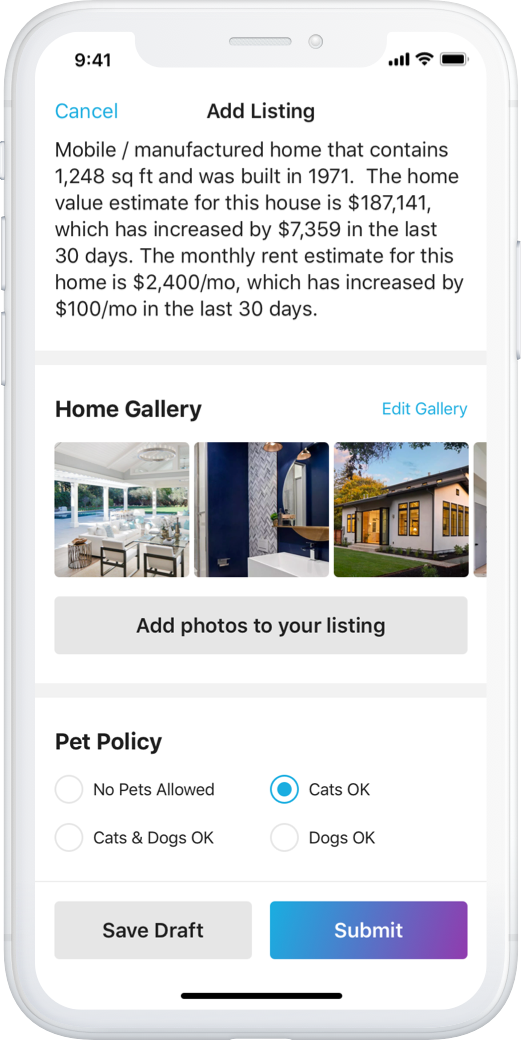The image features a white cell phone displayed against a plain white background, with visible side buttons. The phone's screen shows a mobile interface with a predominantly white backdrop. In the upper left corner of the screen, the time reads "9:41." The upper right corner of the screen displays icons representing cellular signal strength, Wi-Fi connectivity, and battery status.

Directly beneath these icons, the screen displays a blue "Cancel" button on the left and across the center, bold text that reads "Add Listing." Below, there is descriptive text about a mobile/manufactured home. The text states that the home has a floor area of 1,248 square feet and was constructed in 1971. The estimated value of the home is listed as $187,141, an amount that has increased by $7,359 in the past 30 days. Additionally, the estimated monthly rent for the home is cited as $2,400, showing a $100 increase over the last 30 days.

A gray navigation bar follows underneath, displaying "Home Gallery, Edit" on the left side, and "Edit Gallery" in blue on the right side. Below the bar are thumbnail images of three photos of the home, with a fourth image partially visible on the right side of the screen.

Further down, a gray button with black text prompts the user to "Add Photos to Your Listing." Beneath this button, the words "Pet Policy" are written in black font. Below the heading, there are four options each accompanied by a circle: "No Pets Allowed," "Cats and Dogs Okay," "Cats Okay," and "Dogs Okay." The "Cats Okay" option is selected and marked with a blue fill, indicating the current choice.